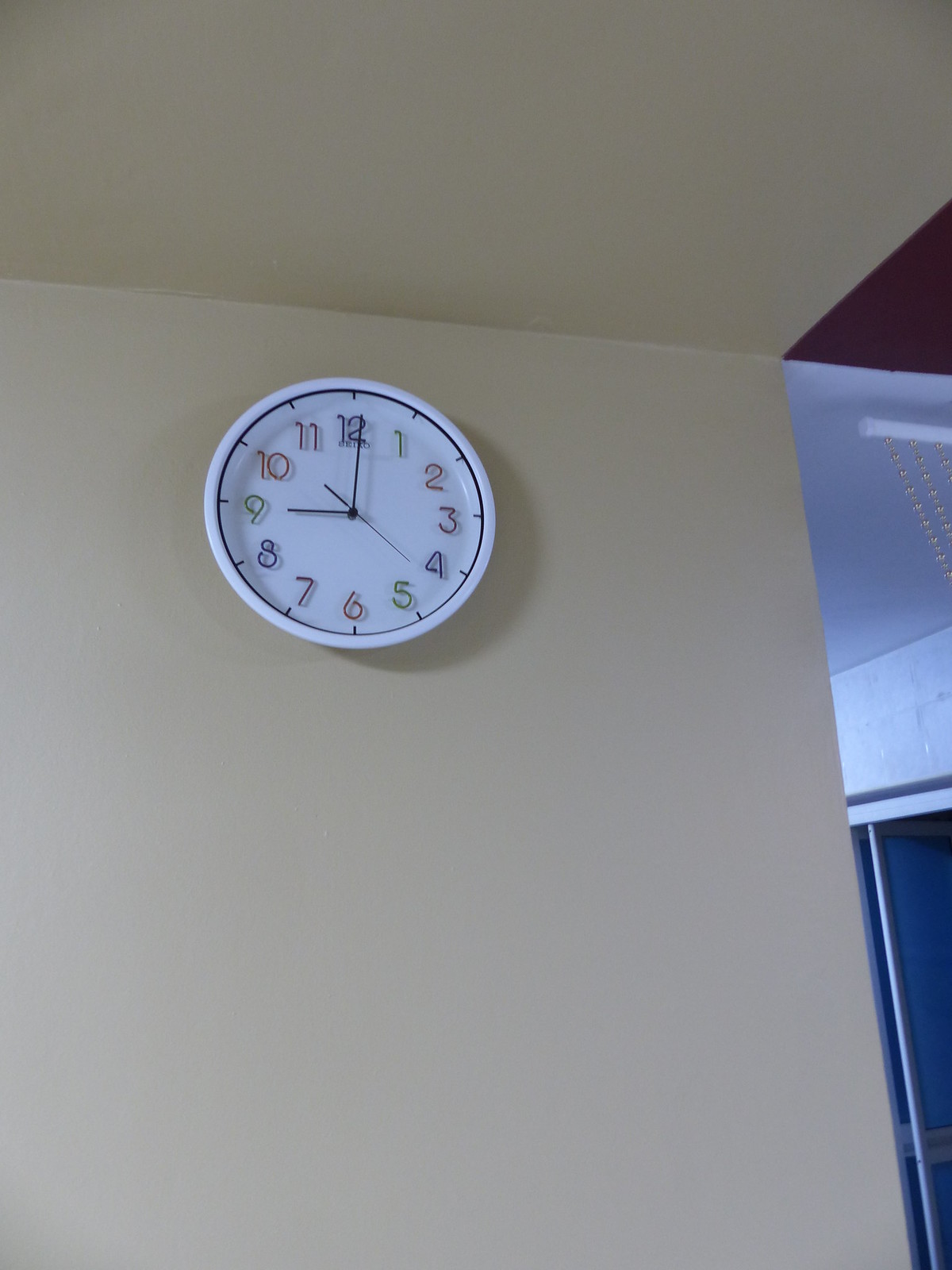This image showcases an interior wall in a house, painted in a light tan color. Mounted high near the ceiling on this wall is a round Seiko wall clock. The clock features a white face with a black border encircling it. The clock's hour markers are uniquely colorful: 12 is blue, 1 is green, 2 is orange or red, 3 is purple, 4 is blue, 5 is green, 6 is orange or red, 7 is purple, 8 is blue, 9 is green, 10 is orange or red, and 11 is purple. The clock hands, including the second hand, are black. To the right of the clock, part of a white ceiling is visible, along with a partial view of what appears to be either a window or a sliding glass door.